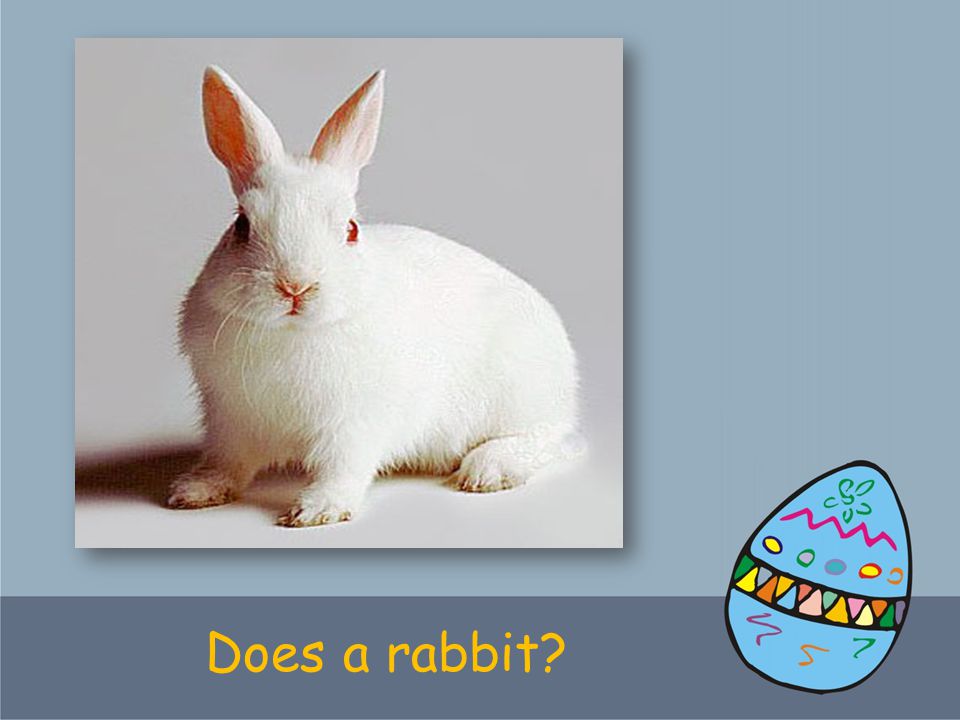This image appears to be an educational slide with a light blue background occupying the majority of the space, and a darker dusky blue band at the bottom. In the bottom band, there is yellow Comic Sans font text that reads, "Does a Rabbit?" To the right of this text, there is an animated blue Easter egg featuring various designs. These include multicolored squiggly lines in shades of purple, orange, and green at the bottom of the egg, and a border of multicolored triangles, incorporating green, yellow, gray, orange, blue, red, and pink. Additionally, there are some decorative dots and a small green flower near the top of the egg. Above this, in the lighter blue section, there is an image of a white albino rabbit with red eyes and upright ears, gazing directly at the viewer. The rabbit is set against a grayish background, enhancing its prominence in the slide.